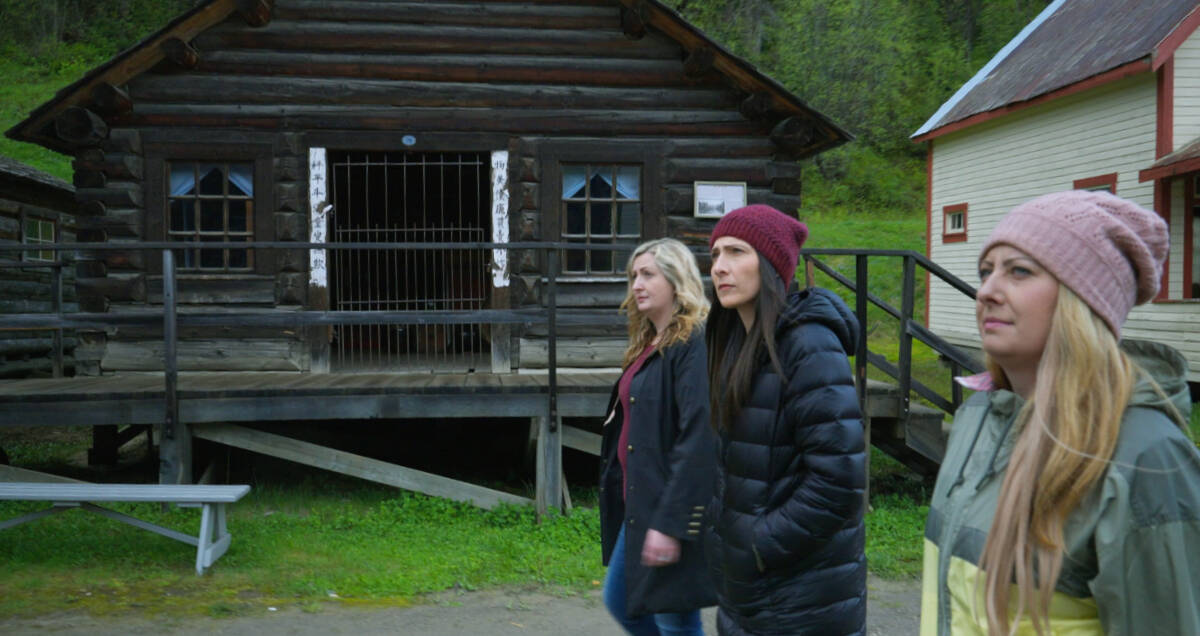Three women, who appear to be middle-aged and white, are walking past a log cabin that looks like a recreated version, with pieces uniformly held together but lacking the traditional connections of an authentic log structure. The cabin is dark brown with a very large iron gate blocking its front doorway, and a wooden rail cordons off the walkway in front. In front of the rise leading to the cabin, there is a light blue wooden bench. To the right, there's a regular house that's light yellow with red details and a brown roof. To the left, another cabin similar to the central one is also visible. The backdrop is densely wooded, suggesting the area is surrounded by wilderness.

The woman in the center of the image has blonde hair with dark roots, wears a dark jacket with long sleeves over a dark red sweater, and has blue pants. To her left, on the viewer's right, is a woman with a burgundy knitted beanie, long dark brown hair, and a puffy black jacket. Her leggings are not visible. Furthest to the right for the viewer, on the left within the group, is a woman with a pale pink knitted beanie, long blonde hair with tan or pink highlights, and a windbreaker-style jacket that is green on top with a dark green center and light yellow-green bottom.